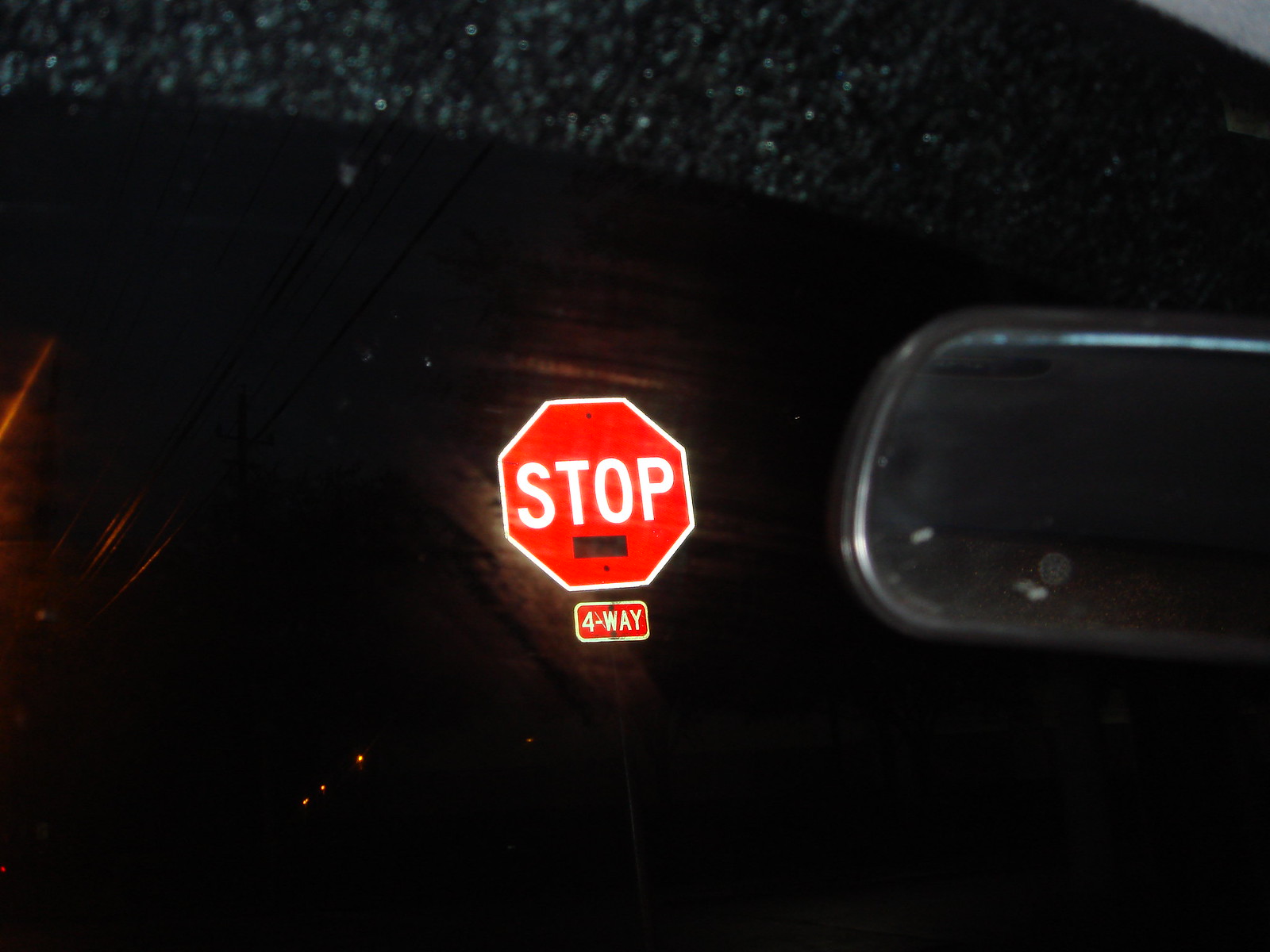A nighttime photograph taken from inside a car captures a vividly illuminated stop sign prominently in the frame, positioned slightly to the right. The red stop sign with bold, white lettering reads "STOP" with "FOUR WAY" indicated beneath it. The illumination provided by the car's headlights starkly contrasts against the surrounding darkness, rendering the stop sign as the focal point. To the right, part of the rearview mirror is visible, adding context to the interior setting of the car. The windshield displays subtle streaks, suggesting either rainfall or accumulated dust, enhancing the texture of the image. In the distance, faint glimmers of headlights add depth to the scene, punctuating the otherwise enveloping darkness.